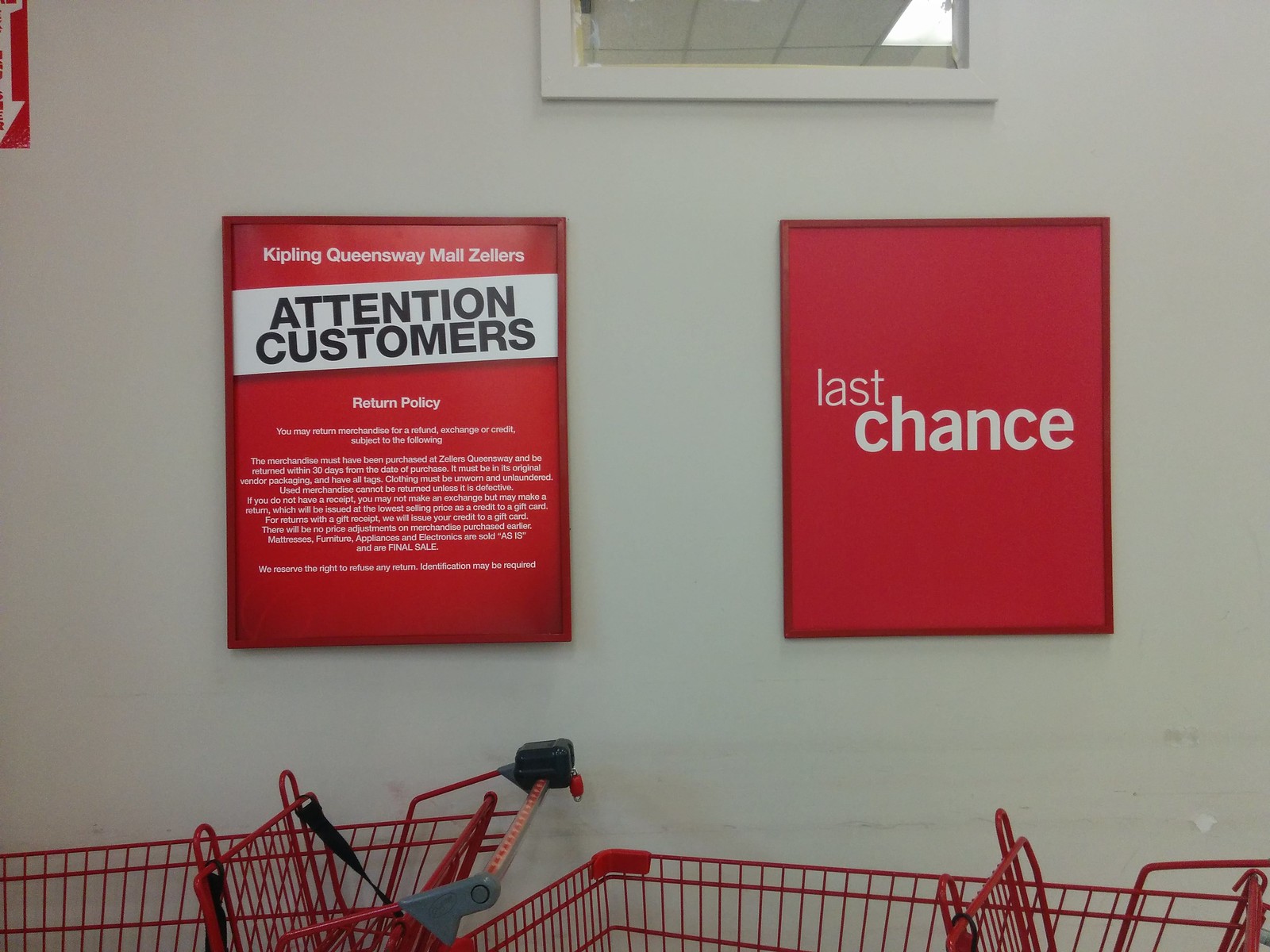This photo depicts a white wall in a store adorned with two framed red signs positioned side by side. The left sign features small print at the top, reading "Kipling, Queensway, Mall, Zellers," followed by a white banner that boldly states "Attention Customers" in black letters. Below it, in very small print, are the words "Return Policy," with a detailed message underneath. The right sign simply states "Last Chance" in white lowercase letters, with "last" positioned slightly above and left-aligned to "chance," which is bolded. Below the signs, the image captures two bright red shopping carts parked against the wall. The cart on the left includes a latch and a seat belt in the basket, indicating it may be designed for a child. Additionally, there is a quarter-operated mechanism for unlocking the carts from one another. In the upper center of the photograph, the bottom of a wood-framed window is visible, matching the color of the wall.